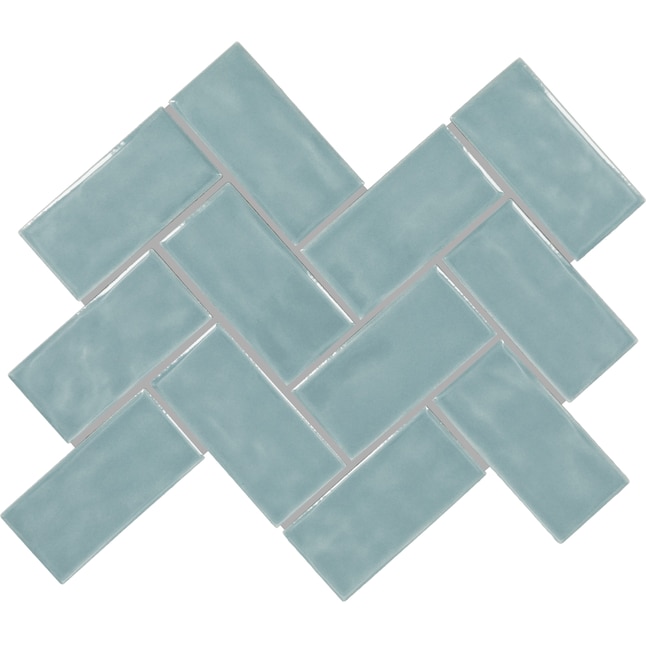The image features a plain white background showcasing a detailed arrangement of small rectangular tiles. These tiles, which are light blue and tan in color and resemble the size of dominoes (approximately half an inch wide by an inch long), are meticulously set in a herringbone pattern. The grout between the tiles is a light gray, enhancing the overall design. Starting from the bottom left, the first tile is angled 45 degrees to the right, followed by another tile positioned 45 degrees to the left, creating the distinctive herringbone effect. This pattern continues upwards for at least three rows, with each tile interconnected at alternating 45-degree angles. The tiles collectively form a broad M shape that can be traced with a finger. The topmost row deviates slightly, with tiles misaligned, adding a unique touch to the pattern.